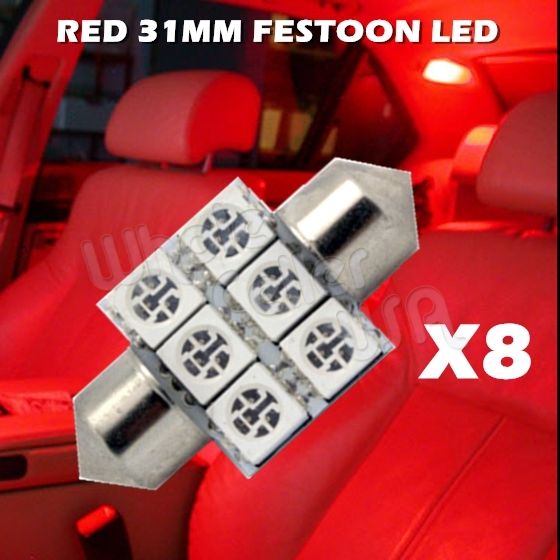This image is an advertisement showcasing a "Red 31mm Festoon LED x8" light. The background features an illuminated red car interior, viewed from a three-quarter angle, revealing the red front seats and part of the seatbelt mechanisms. The car doors are open, casting light onto the back row, where the seatbelts are fastened. Central to the image is the featured product, a 31mm festoon LED cluster. The silver, metal object is shaped almost like a dreidel, comprising a rectangular mounting pad with two rows of three LED elements, flanked by conical ends. The text, in white, prominently displays "Red 31mm Festoon LED" at the top and "X8" on the right, emphasizing the product details. The ad is visually striking, utilizing a red and black color scheme with the metal object prominently overlayed in the center.